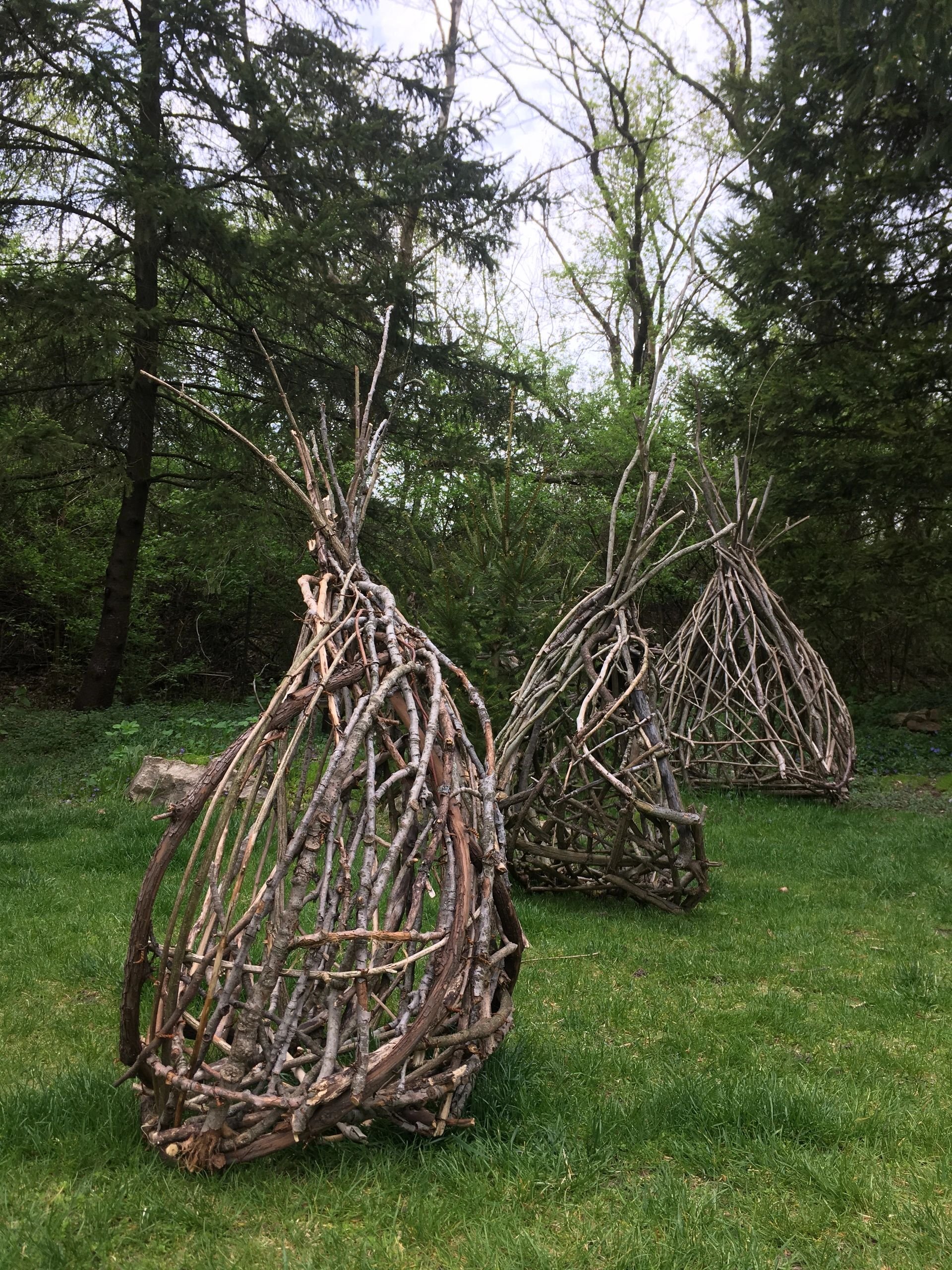This outdoor photograph captures three intricately crafted, pyramid-shaped sculptures made from felled branches, tightly bound together to form structures that are more artistic than functional. These twig-based works of art, resembling large cages or domes, each appear to be filled with additional branches at their bases for added stability. Lined up neatly in a row, the sculptures probably serve as part of an art exhibit. They sit on a grassy field under a blue sky dotted with white clouds, with a backdrop of actual growing trees a short distance away. The day appears slightly overcast, lending a muted brightness to the scene. Despite their substantial size, roughly equivalent to a human's height, the sculptures lack doorways and interiors, affirming their purpose as visual pieces rather than shelters or functional objects.